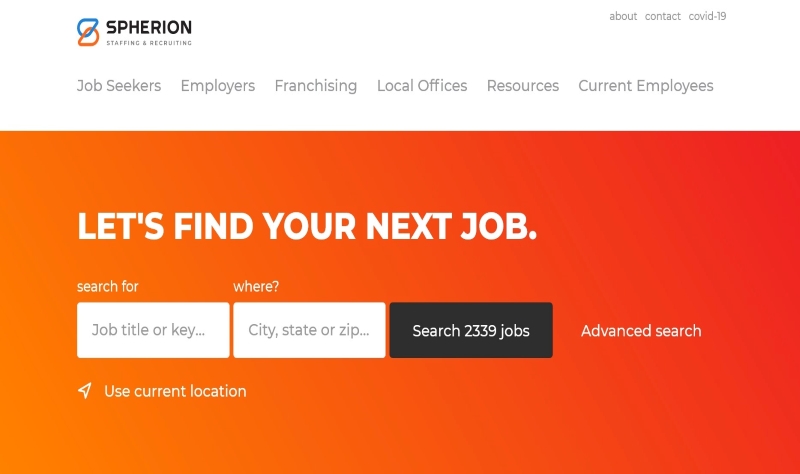The image depicts a screenshot from the job search engine website, Spherion. The Spherion logo is prominently displayed in the top-center, featuring an interlacing design of a blue teardrop turned to the right and an orange teardrop turned to the left, with "Spherion" written in bold black text and "staffing and recruiting" in smaller gray text beneath it.

At the top of the webpage, navigation headings include "About," "Contact," and "COVID-19." Further down, in a secondary navigation menu, are the options for "Job Seekers," "Employers," "Franchising," "Local Offices," "Resources," and "Current Employees."

Centrally located on the page, there is a prominent gradient box transitioning from orange to red. Inside this box, bold white text encourages users with the message, "Let's find your next job." Below this headline, smaller text prompts users to search for a job title or keyword, with fields to input a city, state, or ZIP code. Additionally, users are informed that there are 2,339 jobs available to search through. An "Advanced Search" link is also provided for more detailed job search options, and an arrow pointing to the northeast indicates a feature to use the current location.

Overall, this screenshot gives a comprehensive view of the Spherion job search platform's main interface, designed for seamless navigation and efficient job searching.